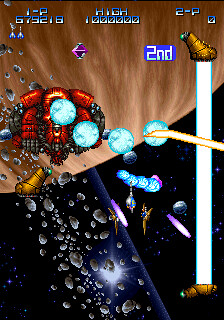The image is a detailed screenshot from what appears to be an old-school, pixelated, 2D game, possibly on a computer or mobile device. The screen is in portrait orientation, displaying various gameplay elements and scores. The top features a scoreboard reading "1P 679,218," and the high score, "Hi 1,000,000," with "2P 0" below it. All text is rendered in a blue-to-white gradient. The background is visually divided; the top half shows a planet set against the blackness of space dotted with stars, while the bottom part is a dark blue. 

Dominating the left is a large creature or space vehicle, characterized by four blue circles—one partially covering what could be its eye. Diagonally scattered across the image, ascending from the bottom left, are grey rocks or meteors. On the right side is a white vertical bar, topped with the word "Second," indicating that it might be player two's turn. Additionally, a small, fairy-like character is seen observing a blue and yellow charm near the bottom of the image. The entire scene is evocative of a chaotic space adventure, with broken rocks and dynamic elements suggesting action within the game.